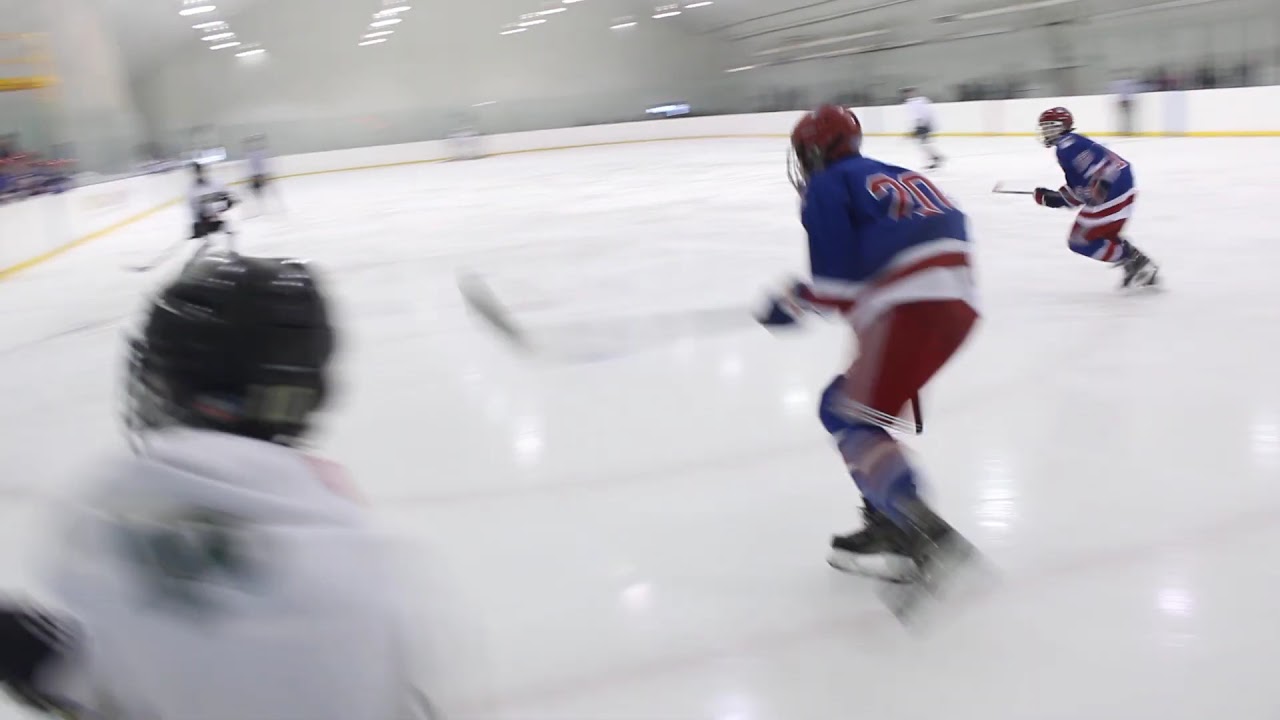The image captures a dynamic ice hockey game taking place on an indoor court with a shiny white surface. The court is encircled by a short white wall, and the ceiling above is white, illuminated by multiple rows of parallel bright lights. In the foreground, two players on the right don blue jerseys and red pants, each accessorized with blue stripes and red helmets. The player closest to the front displays the number 20 on his back, while his teammate, slightly behind, wears number 2. On the left side of the image, three opposing players are visible in white jerseys paired with black helmets. The photograph, taken from the ice rink behind the players, exudes a sense of motion, indicated by a slight blur. Spectators can also be seen standing around the rink, adding to the vibrant atmosphere of the scene. The colors in the image primarily include red, white, blue, black, and yellow. The overall shot effectively conveys the intensity and excitement of an ice hockey match in action.